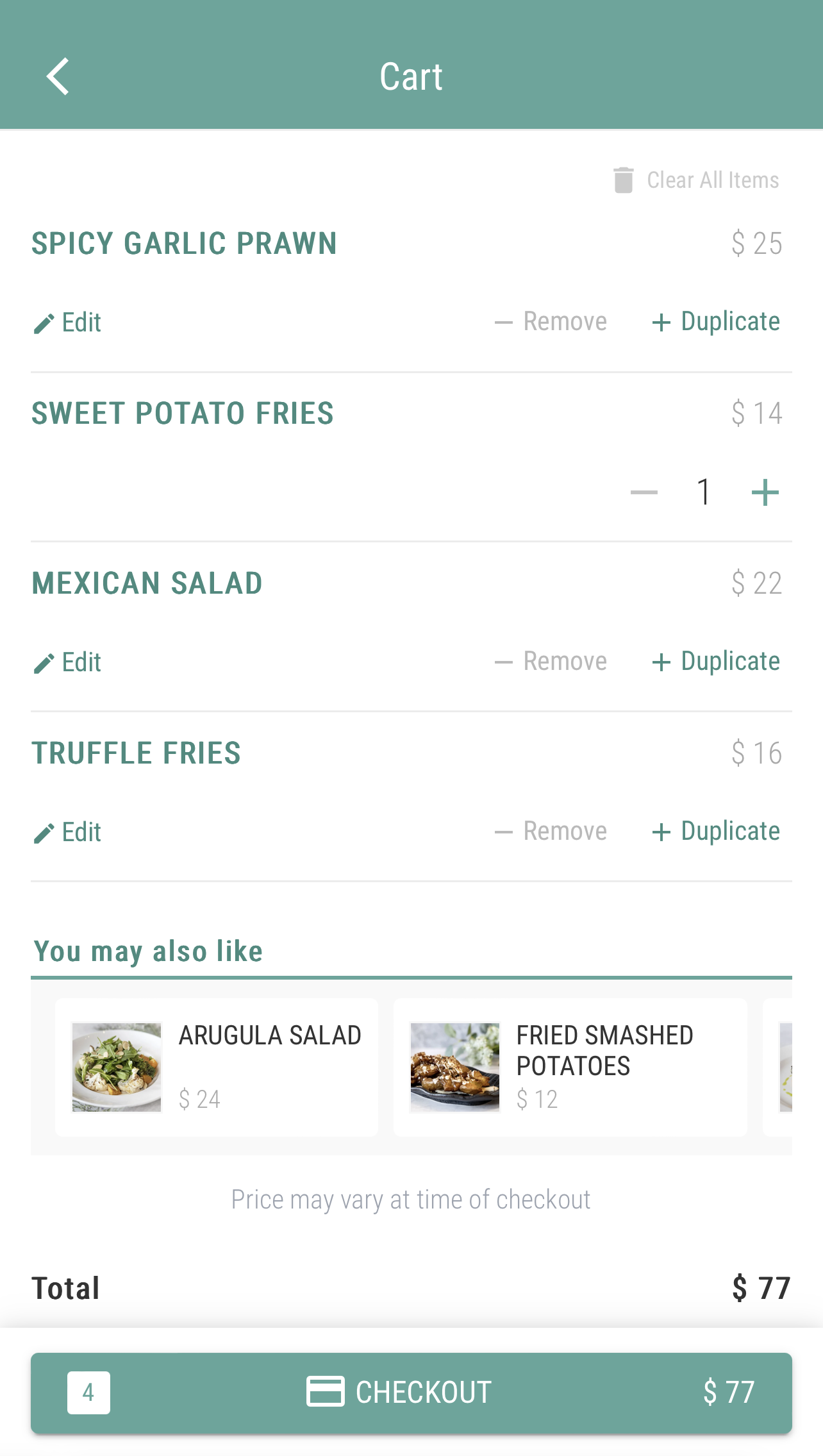At the very top of the image, a long green bar features the word "CART" prominently in white, with each letter separated by dashes (C-A-R-T). On the left side of this bar is a small arrow pointing left. 

Below the bar, in the same green color, it reads "Spicy Garlic Prawn." To the right of this item, approximately three to four inches away, "$25" is displayed in gray text. Below this item, the word "EDIT" appears with a pencil icon beside it, and to the right are options in gray and green: "REMOVE" and "DUPLICATE" (with a plus sign) respectively.

Next, another green item is listed: "Sweet Potato Fries," with "$14" indicated in gray to the right. Below this listing are a series of options for adjusting quantity: a minus sign, the number one, and a plus sign to add more items. 

Following this is the "Mexican Salad," featuring options for "REMOVE" and "DUPLICATE" to the right. Below that is "Truffle Fries," displayed in green like the previous items, with an option to "EDIT" and then to the right "REMOVE" and "DUPLICATE," with a price of "$16" in gray.

Further down, in green and underlined, is the recommendation section labeled "You may also like." This section contains two suggestions: an image of green leaves labeled "Arugula Salad" priced at "$24," and an image of potatoes on a plate labeled "Fried Smashed Potatoes" priced at "$12."

At the very bottom of the image, in a green box, is the word "CHECKOUT" accompanied by the total "$77."